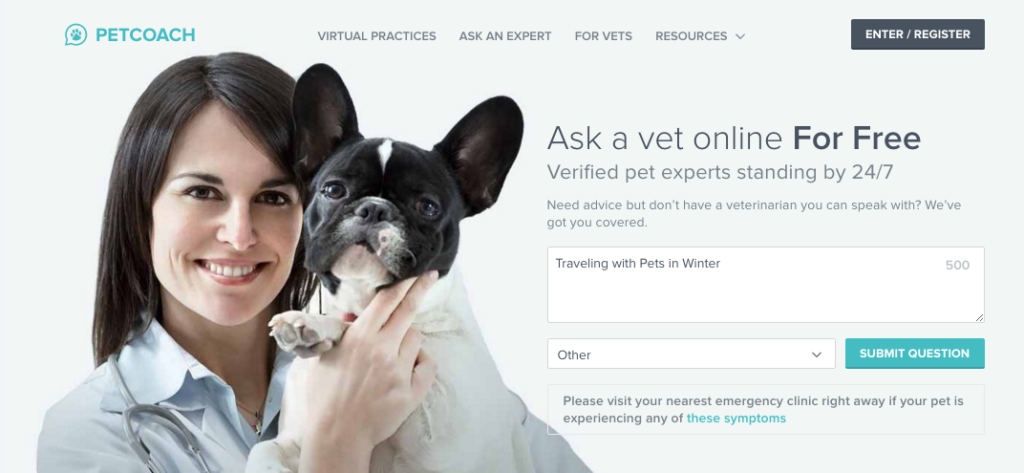The image is a screenshot of the PetCoach website. The PetCoach logo is prominently displayed in green, featuring a paw print enclosed in a circle. The website's navigation menu, positioned at the top, includes the following headers in gray: "Virtual Practices," "Ask an Expert," "4Vets," and "Resources" with a drop-down arrow. On the far right, there is a black box with white text that reads "Enter/Register."

On the left side of the screen, there's a heartwarming photo of a smiling woman holding a small black-and-white dog. The dog has a predominantly black face with a distinctive white streak running down the middle of its forehead, white patches around its whiskers, nose, and chin, and a white body.

Next to the image, there's a bold headline: "Ask a Vet Online for Free, Verified Pet Experts Standing by 24/7." Below this, it says, "Need advice but don't have a veterinarian you can speak with? We've got you covered." A text box labeled "Traveling with Pets in Winter" is visible, with the number "500" on the right side. Directly beneath this, there is a drop-down box marked "Other" and a "Submit Question" button.

At the bottom of the screenshot, a cautionary message urges pet owners: "Please visit your nearest emergency clinic right away if your pet is experiencing any of these symptoms."